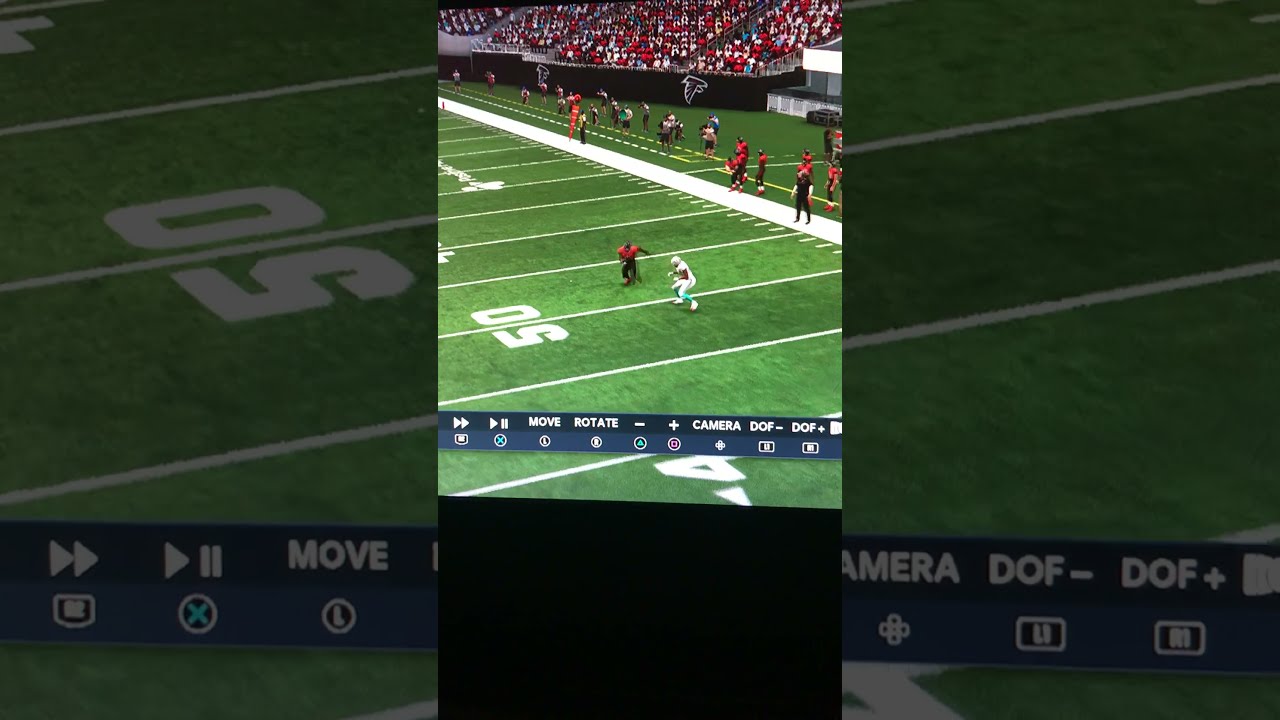This image captures a detailed paused moment from a highly realistic 3D NFL video game, showcasing lifelike players and field details. Centered around the 50-yard line, two pivotal players are locked in action: one in a white helmet, jersey, and light blue pants, resembling a player from the Miami Dolphins, evading a tackle attempt from a player clad entirely in black. Elevating the realism, the sidelines are populated with attentive players, coaches, and staff. The background features enthusiastic Atlanta Falcons fans, predominantly dressed in red and black, enhancing the home game atmosphere. The top of the stands prominently displays the Atlanta Falcons logo. The bottom of the screen is adorned with a functional banner in light and dark blue, offering options for controlling the game view, indicative of a paused game screen. Additional elements include a referee with a marker near the sidelines and the distinct orange yard marker on the green field with white lines. The vertical orientation suggests the screenshot was taken with a cell phone, adding a casual, user-generated touch.